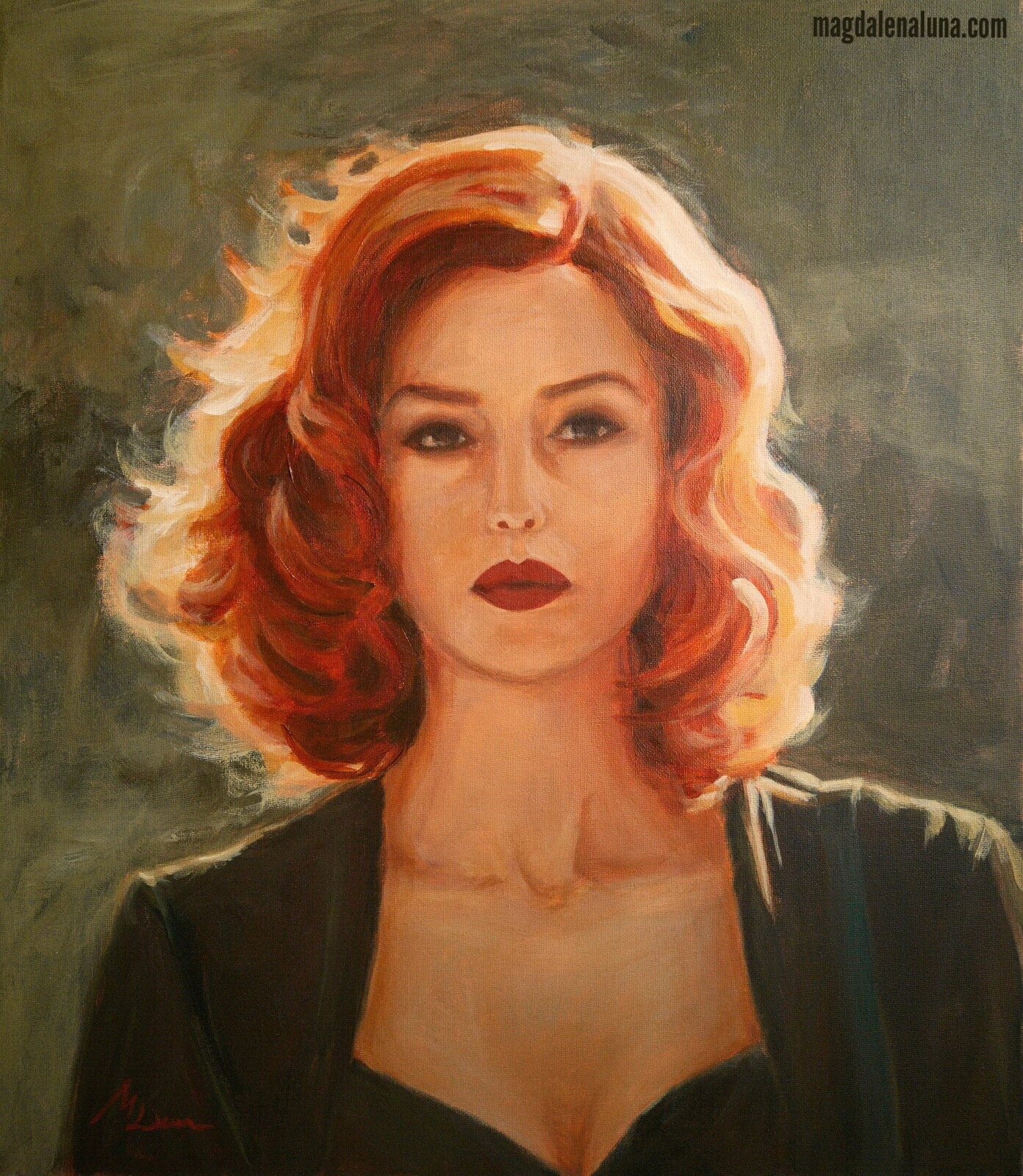This vertically rectangular painting, bordered only by its dimensions, features a digitally added website, magdalinaluna.com, in the upper right-hand corner. Set against a mottled grey and brown background, it depicts a pensive and vividly rendered portrait of a young, attractive Caucasian woman with red, shoulder-length wavy hair. Her wavy hair, rendered with a blondish halo, cascades down to her shoulders, with its hues varying in light and dark. The light in the painting appears to emanate from the upper right, casting nuanced shadows.

She faces the viewer but her gaze is directed upward to the right. Her almond-shaped, brown eyes are accentuated with eyeliner, and her well-shaped eyebrows frame a long, delicate nose. Her peachy white skin and carefully defined neck add to her delicate allure. She wears a dark green, low-cut dress with a matching olive-green jacket, exposing her upper chest and clavicle bones, hinting at a fair amount of cleavage. A blue handbag strap is visible over her shoulder, suggesting a casual, yet poised demeanor. The background intertwines swirls of forest green and white, enhancing the timeless, somewhat haunting quality of the portrait.